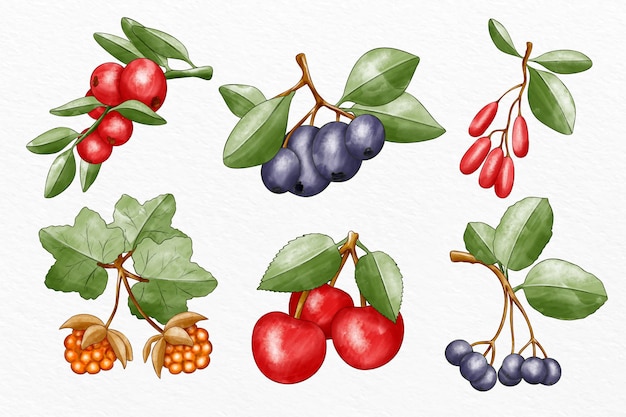This detailed color illustration, in landscape orientation, features a beautiful array of botanical art showcasing six clusters of various fruits. Arranged in two rows of three images each, the top left image displays a blossom of small, round red berries, possibly cherries. The top center showcases a cluster of blue grapes, and the top right features a cluster of oval-shaped red fruits.

In the bottom row, the left image portrays two clusters of golden round fruits. The bottom center highlights three red cherries on stems, while the bottom right exhibits two clusters of blueberries. Each fruit cluster is complemented by meticulously detailed dark green leaves. All illustrations are vibrant and floating on a light gray background, offering a comprehensive and vivid compilation of various berries and fruits.